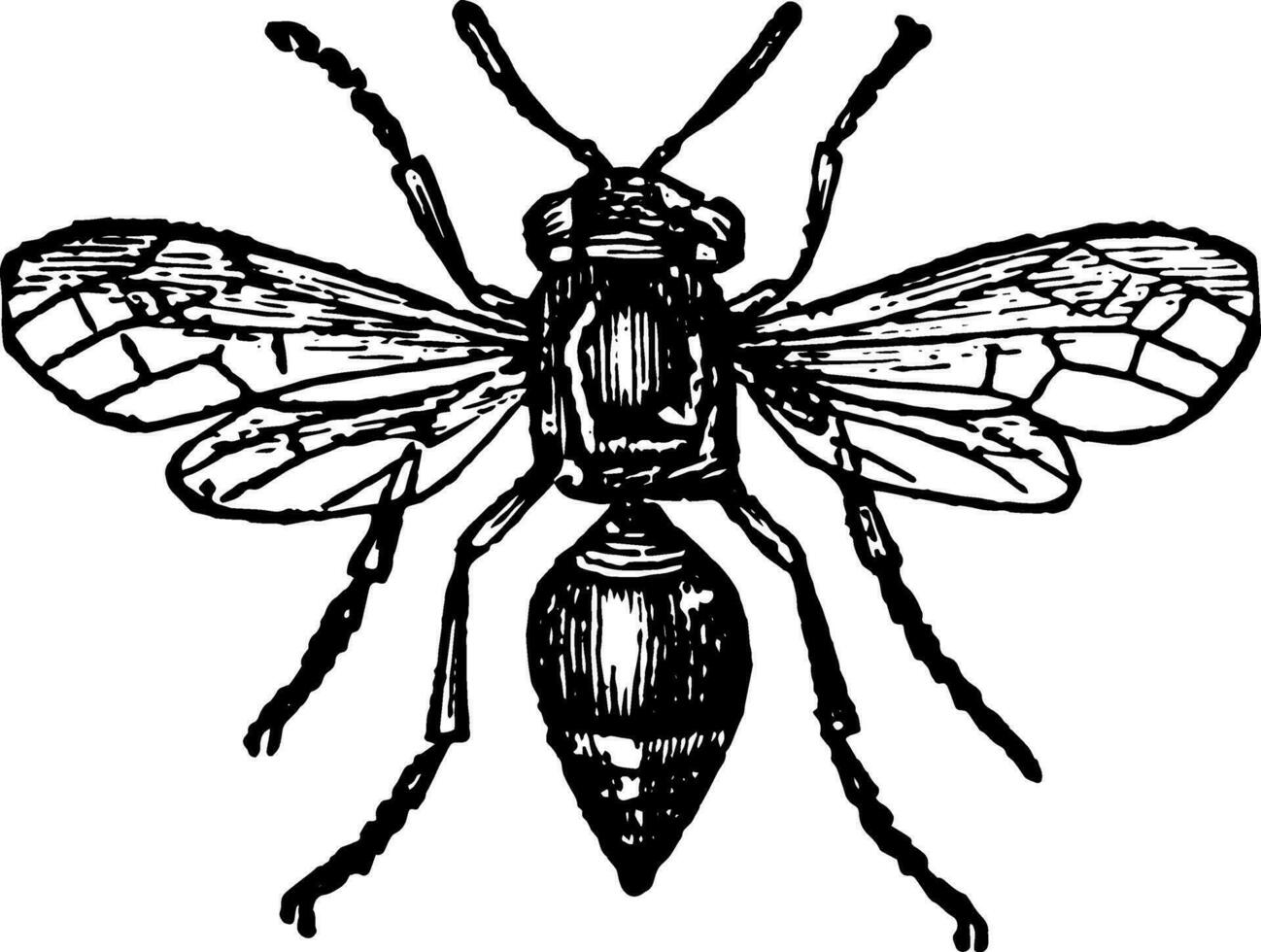A detailed sketch of a housefly is depicted, showcasing intricate features and meticulous details. The fly has a segmented body with three legs on each side, each leg appearing hairy and segmented, terminating in delicate, pointed tips. The torso is square-shaped with a distinctive body structure that transitions into a bulbous lower body reminiscent of a Christmas ornament – rounded at the top and tapering to a diamond-shaped end. The head of the fly is stark white, adorned with large, expressive eyes similar to those of the Pokémon Bulbasaur. Extending from its head are two antennas that jut out in opposite directions. Its two pairs of clear wings are delicately drawn with black markings that accentuate their transparency. The fly's pose includes some legs raised alongside the antennas, adding a dynamic element to the sketch. The entire drawing is set against a pure white background, creating a stark contrast that highlights the fly’s detailed anatomy.